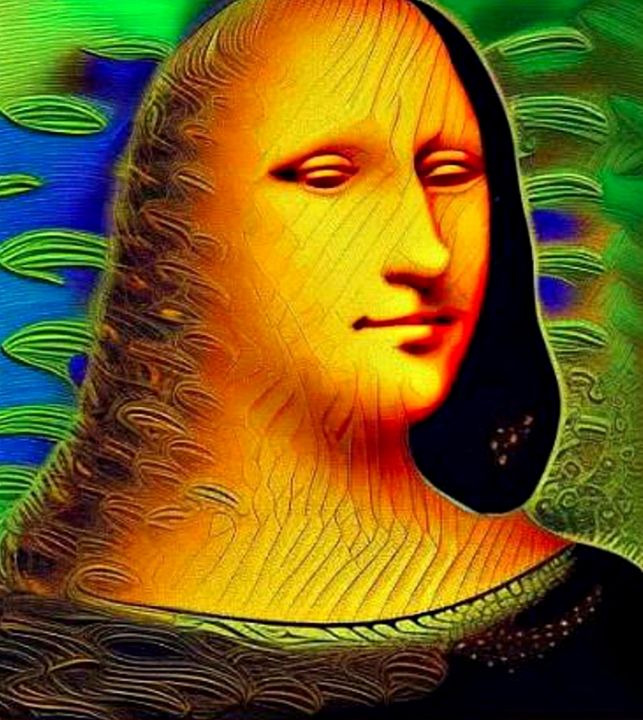This image appears to be a highly stylized and psychedelic 3D manipulation of the Mona Lisa, created through various filters, potentially including AI. The iconic expression and garb are retained, but transformed with unique artistic elements. Mona Lisa’s skin is depicted with an intriguing texture, resembling cracked paint or scales, particularly noticeable on her right cheek. Her face is predominantly orange with bright red shadows, giving it a monochrome, posterized effect.

The right side of her hair looks almost like a void, with minimal texture except at the bottom. In contrast, the left side of her head is adorned with odd, swirly patterns that seem to melt in and out of her hair, adding to the image’s surreal quality. Behind her, the background features a striking green and blue fractal design, with blue-dominant patterns on the left side and green ovals swimming over a green background on the right. These elements create an overall psychedelic effect, reminiscent of peacock plumage, and add to the otherworldly aura of the piece. The combination of these superimposed images and vibrant colors gives the artwork a unique, almost otherworldly twist while still retaining the essence of the Mona Lisa.